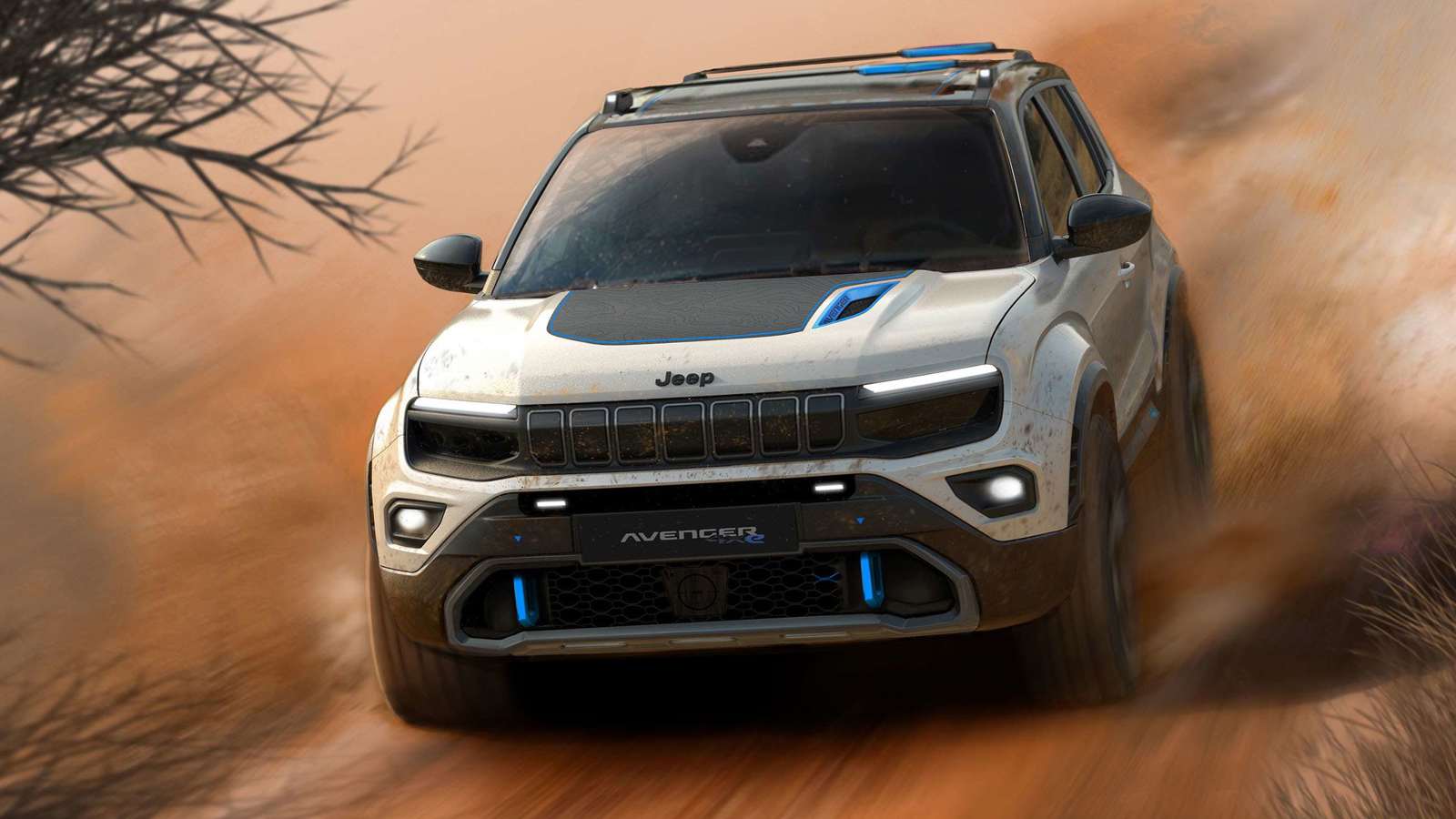The image showcases a sleek, modern Jeep SUV speeding through a desert-like landscape characterized by its reddish clay terrain, subtly accented with patches of white in the background. The SUV, central to the image and slightly blurred around the edges to convey motion, is distinctly silver with black accents around the grille, tires, and base. Adding to its contemporary design, blue accents are visible on the fog lights, ski rack, and one spot on the hood. The vehicle proudly bears the "Jeep" branding in black lettering on the hood, with "Avenger" inscribed beneath the black grille in grey letters. The blurred terrain enhances the sense of speed, and the vague, leafless branches in the upper left corner frame the dynamic scene.